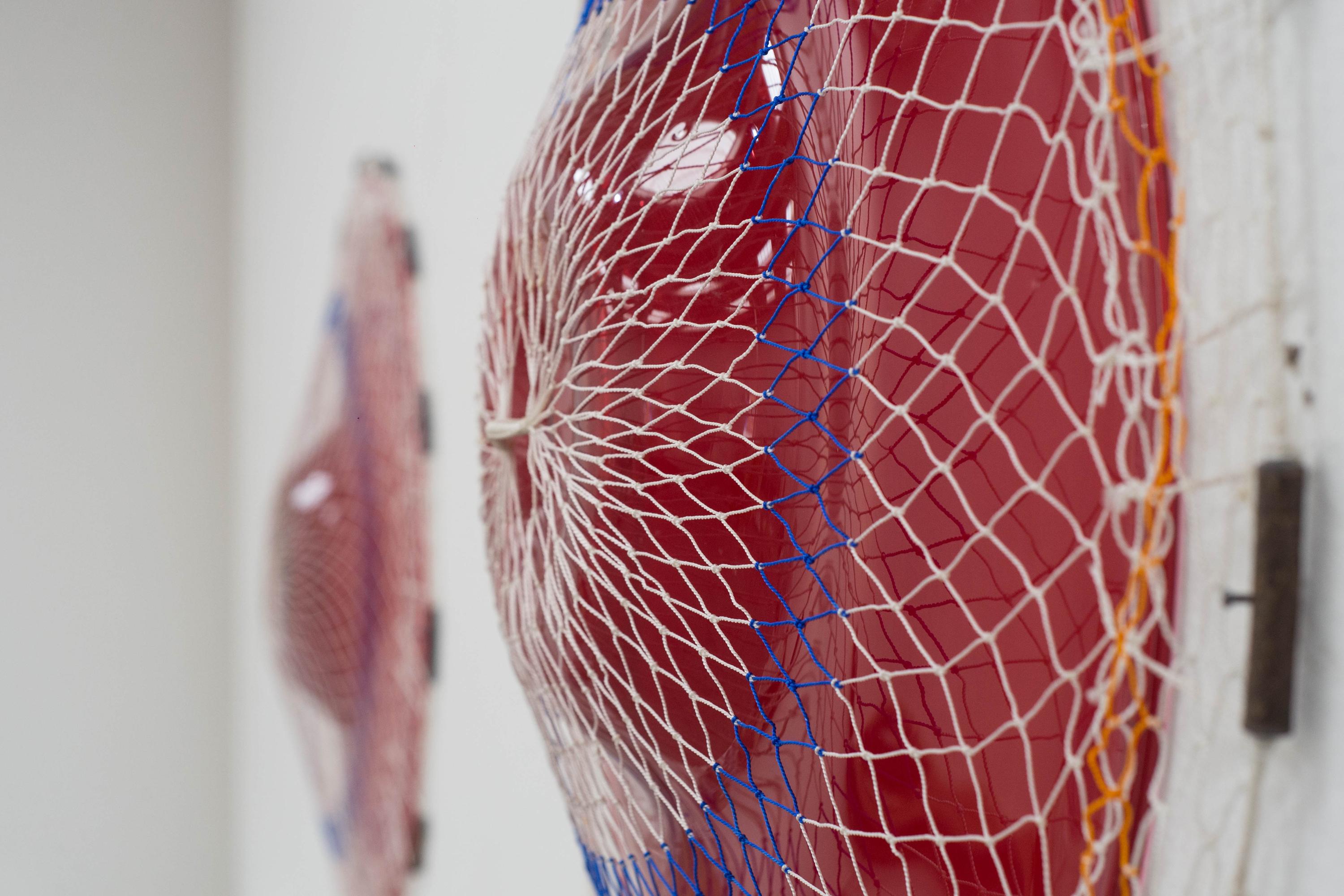The image is a horizontally rectangular photo of two red, round metal bells mounted on a white wall. Both bells are adorned with a white netting featuring cross patterns, with a distinct blue cross where the net meets the side of each bell. The bell in the foreground is more clearly visible, highlighting its shiny metal surface and a silver knot on top. The second bell, situated further down the wall, appears blurry but reveals similar characteristics. A black latch is visible on the right edge of the image. There's a noticeable white circle of reflected light on the front bell and a hint of orange color where the netting ends on this bell. The overall palette includes shades of pink, purple, white, orange, green, and gray.